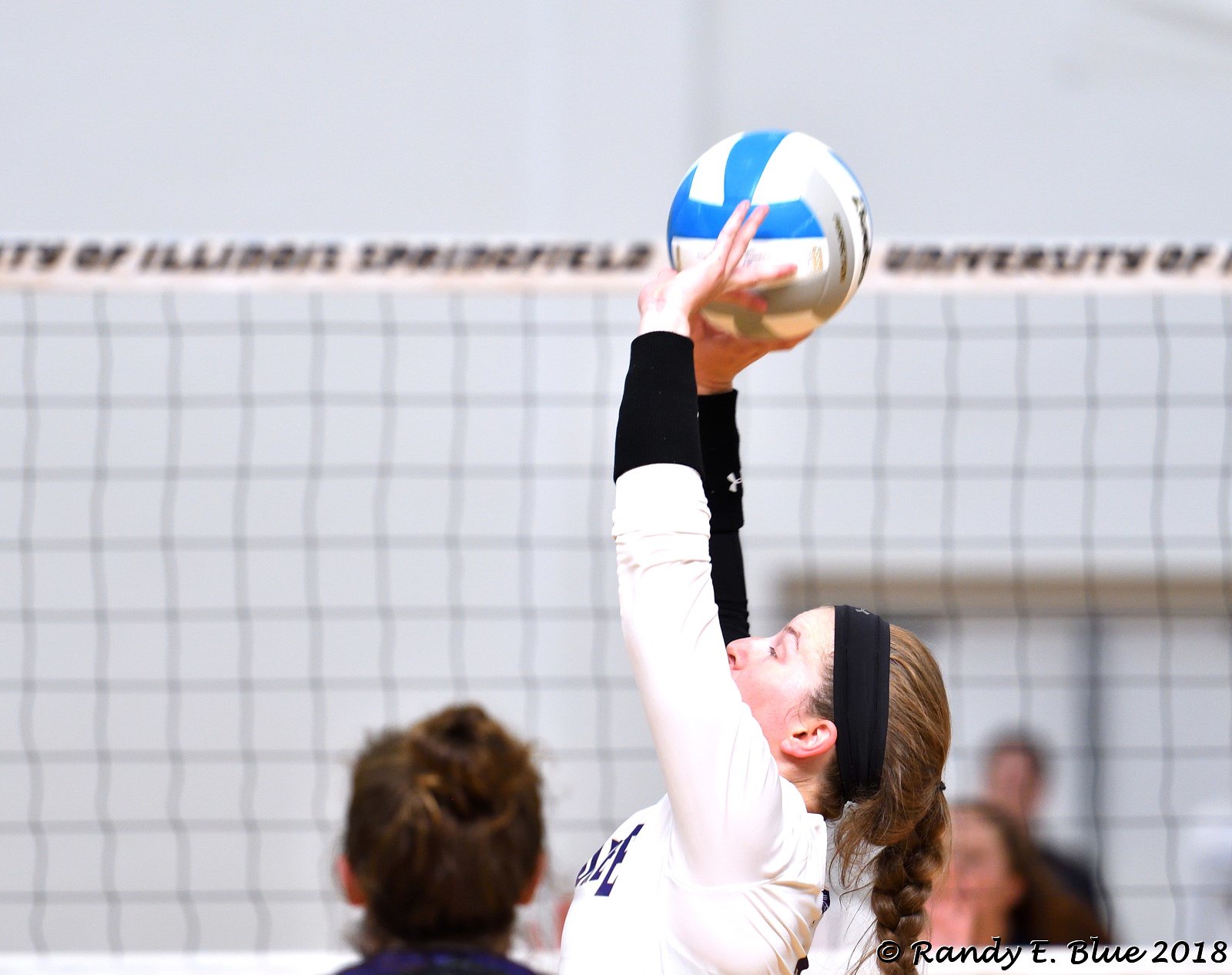In this detailed image captured by Randy E. Blue in 2018, a female athlete from the University of Illinois Springfield is seen playing volleyball. The main focus is on a girl in mid-motion, about to spike a blue, gray, and white volleyball over the net, which prominently features the text "University of Illinois, Springfield." She wears a white uniform with a black undershirt and a headband, her hair styled in a single French braid down her back. Positioned almost at the center of the frame, she appears to be the central figure. Other players are visible but mostly indistinct, with some partial views of their heads and bodies seen around the edges. The scene takes place indoors during a volleyball match, where the background includes additional players and parts of the venue. The environment is accented with colors like gray, white, blue, silver, black, and brown. The image carries a clear copyright mark, noting "Copyright Randy E. Blue 2018" in the bottom right corner.